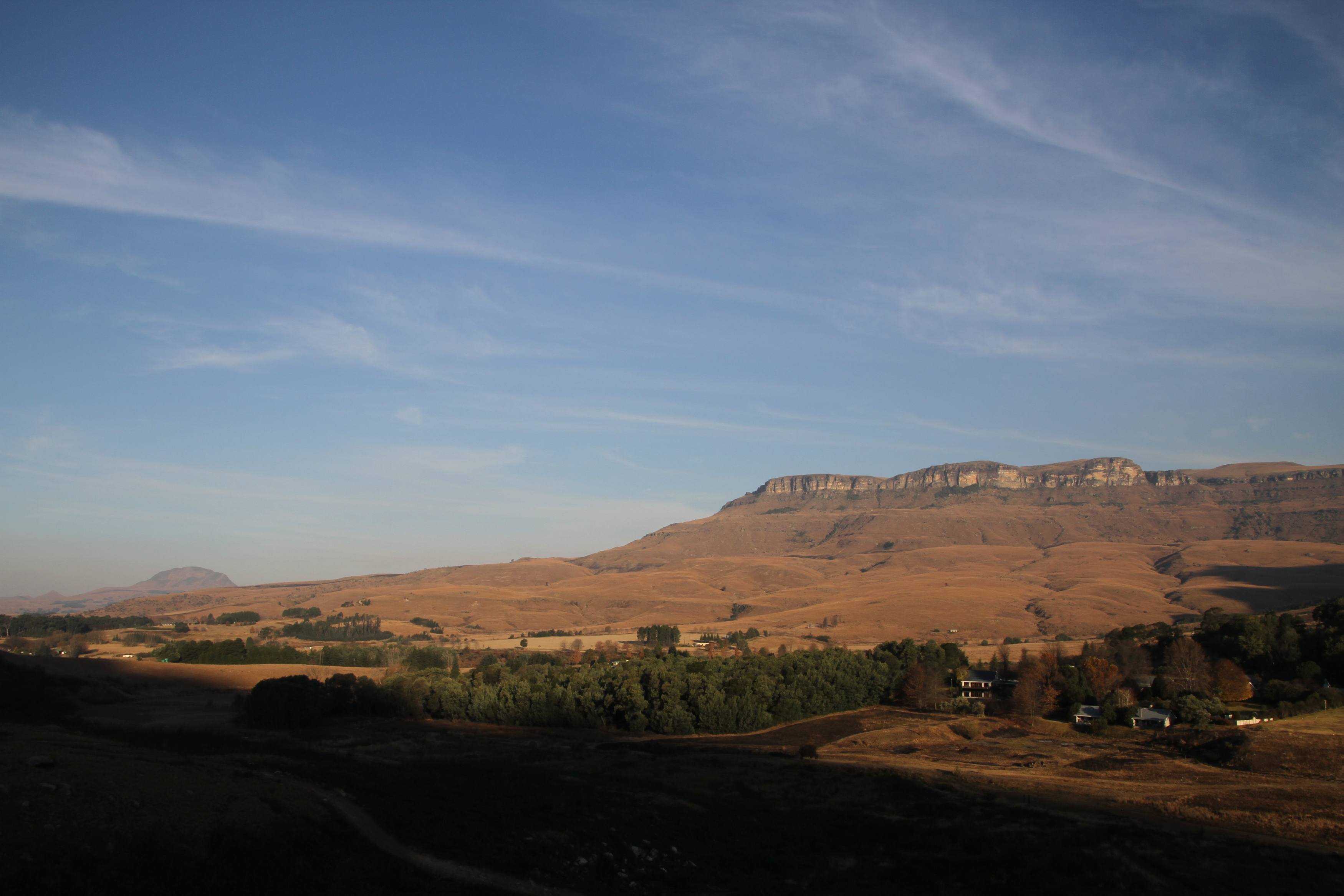The photo captures a vast, open landscape reminiscent of the Utah countryside. Dominated by reddish-brown sandstone formations, the scene transitions from rounded, rocky outcrops to rugged cliffs with distinct ridges and rounded tops. In the lower center foreground, there is a cluster of dark green trees, contrasting with additional brownish trees more towards the right. A small river or stream appears to wind through this area, adding an element of water to the otherwise dry scene. The lower left portion of the image is dark, potentially indicating an obstructed view from within a vehicle or some other shadowed source. The sky overhead is a pale to medium blue punctuated by wispy, whitish clouds. A vehicle is visible on a road to the right, and two or three small homes are nestled inconspicuously among the green shrubbery and trees, blending into the expansive, hilly terrain. The landscape is characterized by its open fields and dirt roads, with the dominant color palette being varying shades of brown and green.